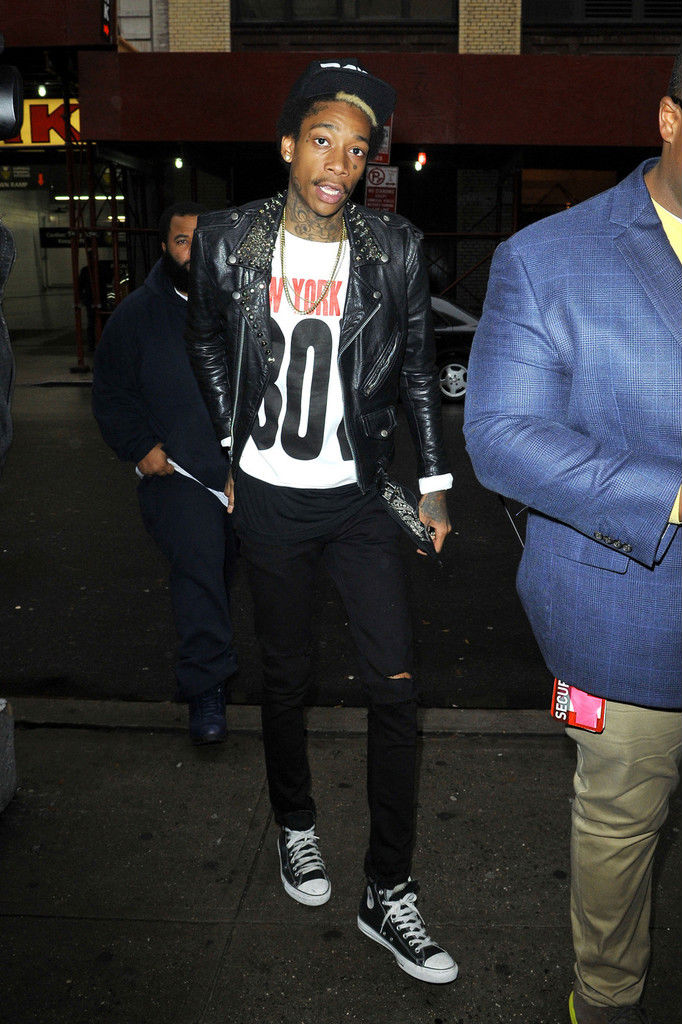This image features the rapper Wiz Khalifa prominently centered in the frame. He appears to be surprised as he looks directly at the camera, mouth partly open and showing his white teeth. Wiz Khalifa is wearing a black leather jacket with studded lapels over a white t-shirt that partially reads "New York, 8-0 something." His shirt is slightly obscured by the jacket. He also has on skinny black jeans that are ripped at the knee and black and white Converse sneakers with white laces. His outfit is accessorized with a black baseball cap, tilted slightly backward, and one or two gold chains around his neck, revealing some of his neck tattoos. His hair is a blondish-blue hue. 

In the foreground, a man is standing slightly to the right, wearing a quilted-pattern blue blazer, a yellow shirt, khaki pants, and a red badge at his waist that reads "SECURITY." Behind Wiz Khalifa is another man dressed entirely in black, partially obscured by Wiz's right shoulder. The scene appears to be outdoors at night, enhancing the dramatic lighting of the photograph.